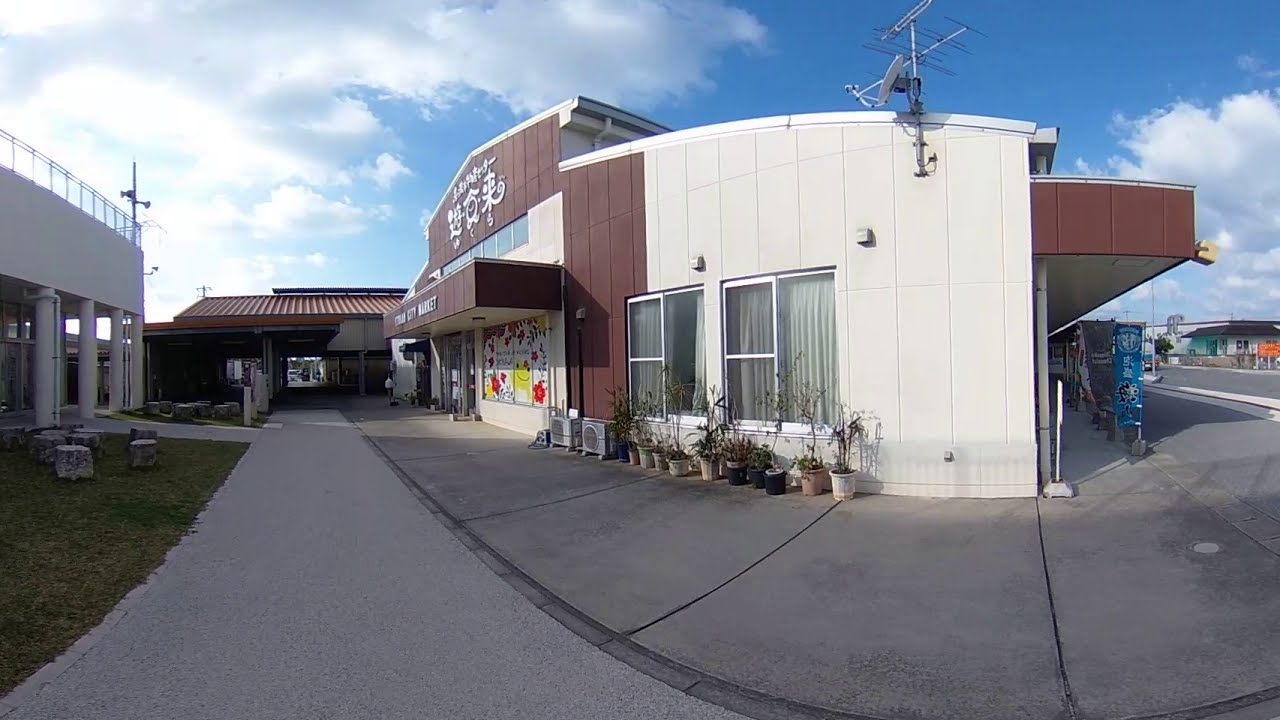The image captures a vibrant suburban area that seems to be somewhere in Japan, evident from the Asian characters on the building. Dominating the scene is a market, possibly specializing in Asian goods, adorned with enticing colors like yellow, red, and white to attract patrons. The market's signage includes something city market and has Asian characters near the roof. To the left of the market is a parking structure, while to the right, there's a blue banner on the sidewalk. Across from the market is a building that might belong to the Knights of Columbus, featuring columns and a red roof or tower. The street on the right side is flanked by a walking path on the left, lined with numerous planters filled with vibrant plants and flowers. The scene is framed by a clear blue sky dotted with puffy white clouds, adding to the picturesque suburban setting. In the very back, there’s a roof over another structure, possibly a garage or an extension of the Knights of Columbus building.